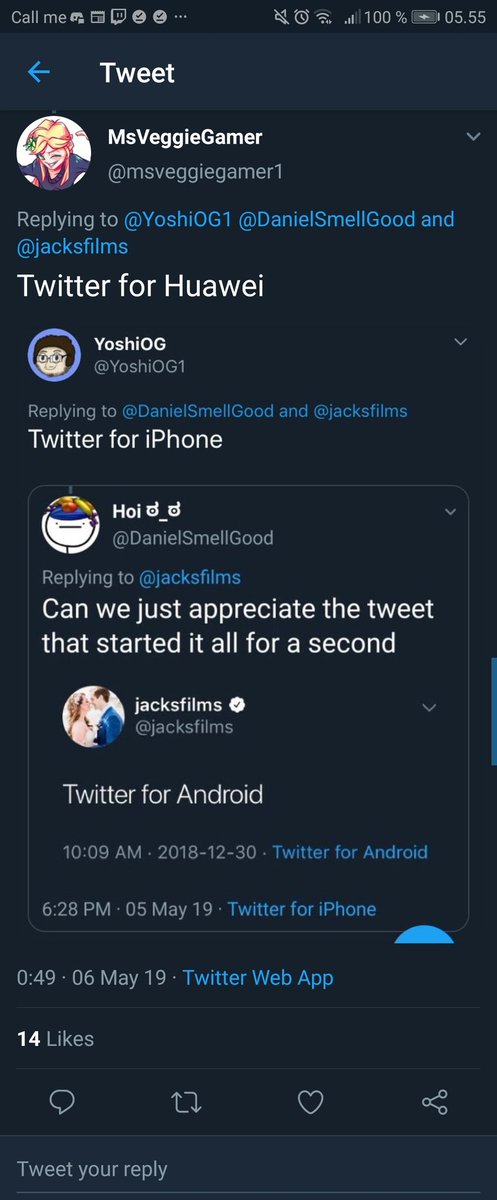In the image, a person uses their smartphone to browse Twitter. The phone screen displays a detailed view of a Twitter conversation thread. 

At the top of the screen, a status bar indicates full battery with a 100% charge and the current time is 5:55. Various notification icons are present, divided by a gap with more icons aligned to the right. The words "call me" appear prominently.

A blue left-pointing arrow labeled "Tweet" is situated beneath the status bar, signifying a new tweet prompt. Below this, a user named MsVeggieGamer, with the handle @MsVeggieGamer1, is replying to other users: YoshiOg1 (@YoshiOg1), DanielSmellgood (@DanielSmellgood), and JacksFilms (@JacksFilms). Notably, the tweet indicates "Twitter for H-U-A-W-E-I," emphasizing the misspelling of Huawei.

Following this, YoshiOg (@YoshiOg1) is also seen replying within the same thread, using "Twitter for iPhone." A subsequent reply in the thread reads, "Can we just appreciate the tweet that started it off for a second?" identified as being sent from "Twitter for Android."

Throughout the conversation, time stamps and device indicators (Twitter for Android, Twitter for iPhone) are dispersed. At the bottom area of the screen, indicators show "14 likes" along with options like "Tweet your reply," accompanied by several functional icons.